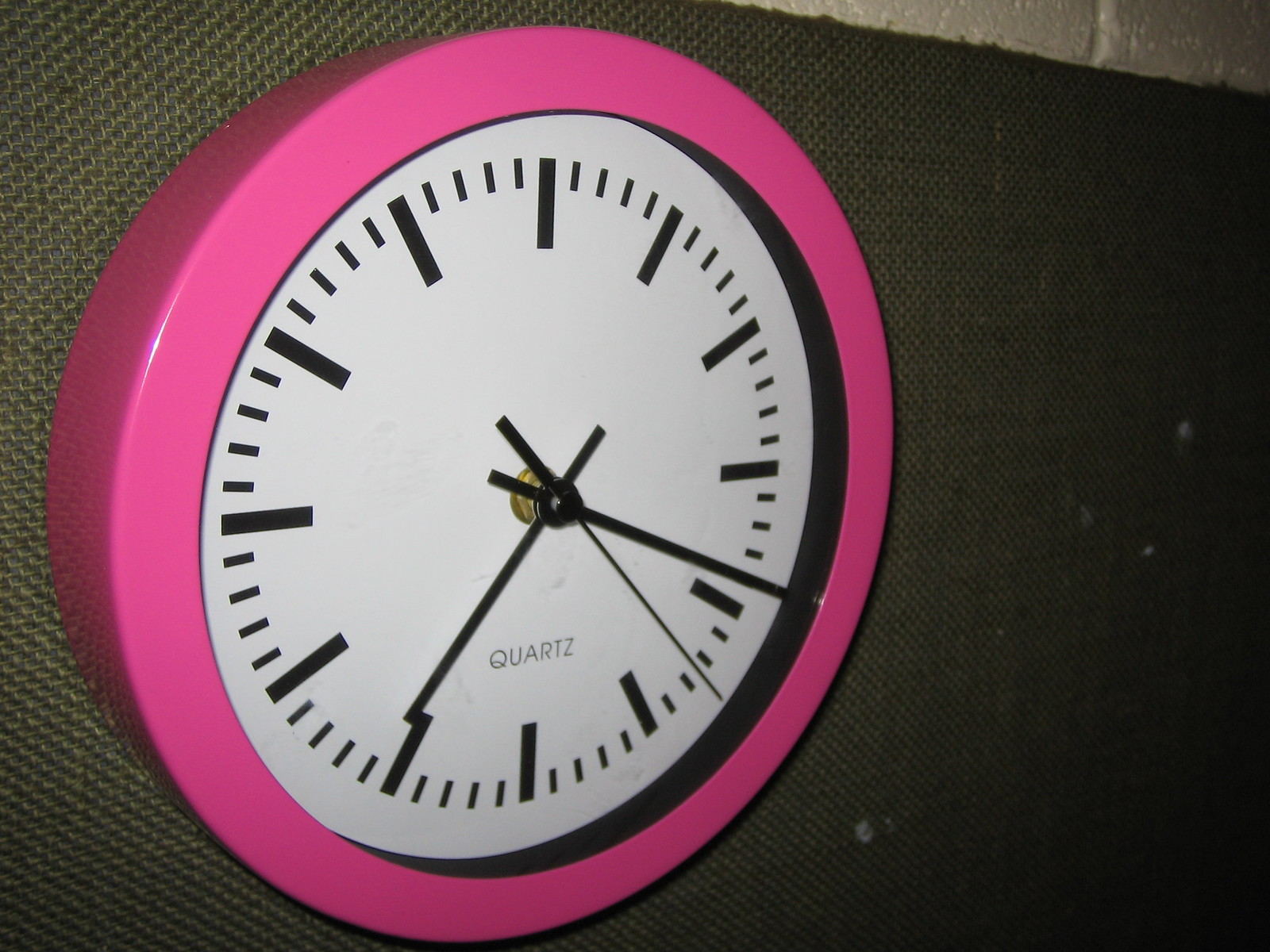The image showcases a vibrant hot pink plastic clock hanging against a rough, unfinished wall. The clock features a prominent hot pink outer rim framing a white face. Instead of numbers, the clock face is marked by thick, long lines at the hour positions and shorter lines in between. The time displayed is 7:19, indicated by simple, sleek hands. A thin black second hand is also visible. The inner edge of the clock face is accentuated by a black trim. The clock is mounted on a piece of burlap fabric, which has noticeable white stains, adding a rustic contrast to the bright, modern clock design. The unfinished wall in the background adds an additional layer of texture and depth to the overall scene.